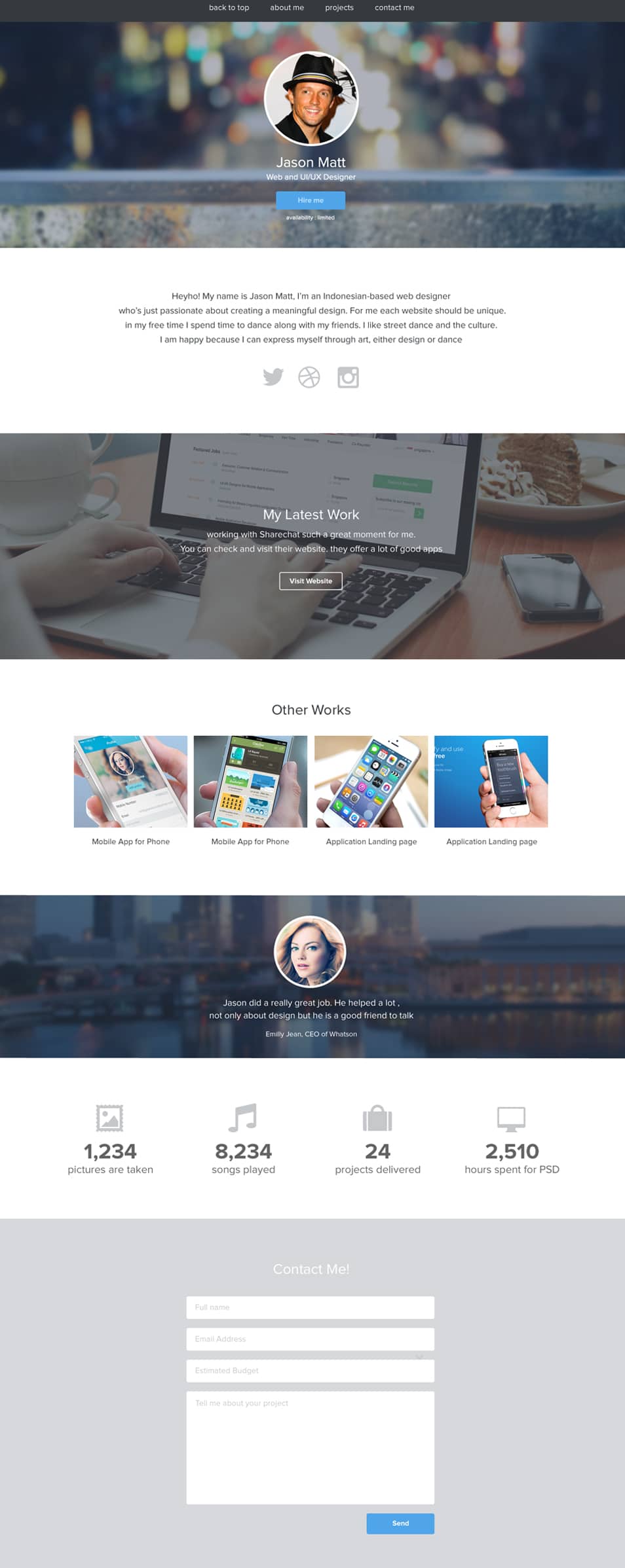This is a detailed screenshot of a personal portfolio website belonging to Jason Matt, a web and UI/UX designer based in Indonesia.

### Top Navigation Bar:
The website features a gray top navigation bar with white text links: "Back to Top," "About Me," "Projects," and "Contact Me."

### Hero Section:
In this section, there is a photograph of Jason Matt—a white man wearing a black fedora hat and a black shirt. Accompanying the photo is a brief introduction: "Name's Jason Matt, web and UI/UX designer." A prominent blue button with white text reads, "Hire Me," followed by a note on his limited availability.

### Background Imagery:
The background displays a blurred image of a city at night, creating a dynamic and engaging atmosphere.

### About Section:
Below the hero section, Jason introduces himself further:
>"Hey-ho, my name is Jason Matt. I'm an Indonesian-based web designer who's passionate about creating meaningful design. For me, each website should be unique. In my free time, I spend time dancing with my friends. I like street dance and the culture. I am happy because I can express myself through art, either design or dance."

### Social Media Links:
Three icons representing old Twitter, basketball, and old Instagram logos are displayed, providing easy access to his social media profiles.

### Featured Work:
A section showcasing someone typing on a laptop, accompanied by text that reads:
>"My latest work, working with ShareChat, such a great moment for me. You can check and visit their website. They offer a lot of good apps," along with a button to view the website.

### Portfolio:
This section highlights several of Jason's projects, including:
- A mobile app for iPhone
- A mobile app for non-iPhone devices
- Two different application landing pages

### Testimonials:
Displayed is a testimonial with a scenic background of a city by a lake and the headshot of a blonde white woman. The testimonial reads:
>"Jason did a really great job. He helped a lot. Not only about design, but he's a good friend to talk to." 
- **Emily Jean, CEO of Watson**

### Statistics:
Jason lists some impressive statistics:
- 1,234 pictures taken
- 8,234 songs played
- 24 projects delivered
- 2,510 hours spent on PSD (Photoshop design)

### Contact Form:
At the bottom of the page, there is a contact form asking for:
- Full Name
- Address
- Estimated Budget
- Details about the project

A "Send" button enables users to submit their inquiries.

Overall, this website serves as Jason Matt’s digital portfolio to showcase his work and attract potential clients.